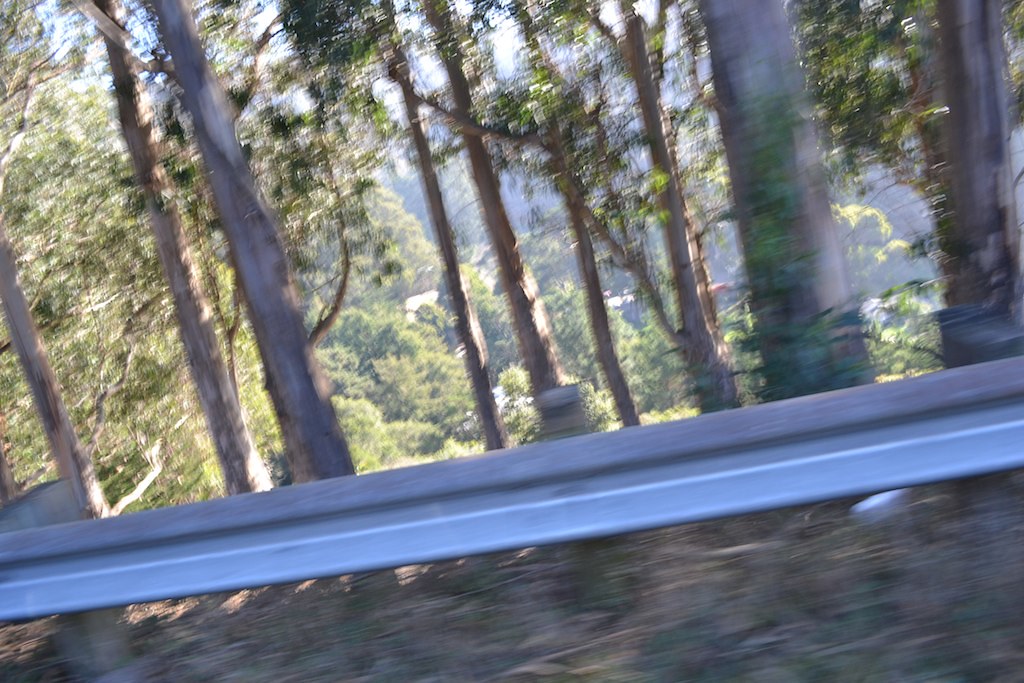This is a blurry color photograph, likely taken from a moving car, depicting a horizontal, rectangular scene. Starting from the lower left corner and extending to the middle of the right side, a silver guardrail is visible. This guardrail runs parallel to what seems to be a roadside, suggesting its purpose is to prevent vehicles from veering off due to the high cliff visible in the background. 

Beyond the guardrail, the ground appears to be a mix of dirt, green patches, and tan or yellow grass. Sunlight filters in from the top left corner, illuminating some of the nearby trees. The trees' trunks are varied in thickness; some are thin and tall, while others are thicker. These trees are likely birch, with green leaves and occasional sunlight giving them a shimmering effect. 

Further off in the distance, past the initial row of trees, more trees can be seen, possibly on a mountain or in a valley. A small patch of blue sky is visible, indicating it was a sunny day. The blurriness of the image gives it a sense of motion, reinforcing the idea that it was taken from a moving vehicle.